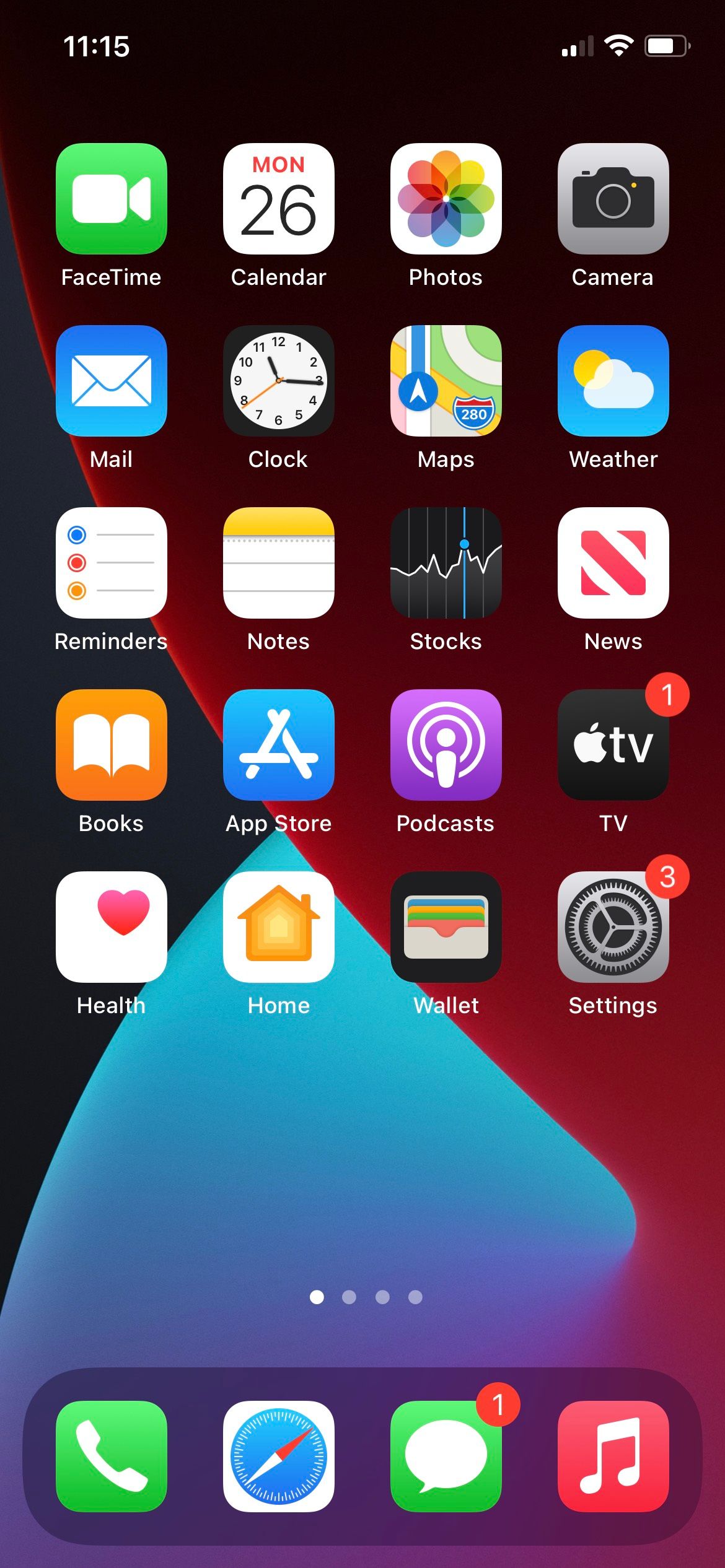Screenshot of an iPhone home page featuring a grid layout of app icons against a modern, geometric background. The background includes a blue gradient overlapping with a red diagonal, circular section, and a black area on the left, resembling two intersecting spheres.

In the top left corner, the time is displayed as 11:15. The top right corner shows two out of four cell signal bars, full Wi-Fi signal strength, and a battery at approximately 75% charge.

The home screen has a 4-column grid layout of various apps, listed as follows:
- FaceTime
- Calendar
- Photos
- Camera
- Mail
- Clock
- Maps
- Weather
- Reminders
- Notes
- Stocks
- News
- Books
- App Store
- Podcasts
- Apple TV

Some apps have notification badges: a red circle with the numeral '1' for updates or notifications and a red circle with the number '3' for other updates further down.

On the final row of apps:
- Health
- Home
- Wallet
- Settings

At the bottom, there are four vertically oriented dots with the leftmost dot highlighted in white, indicating that this is the first page out of four. The fixed applications at the bottom, present on all pages, include:
- Call app
- Safari
- Messages (with a red circle indicating one unread message)
- Music